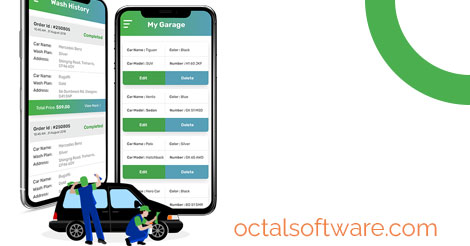This image features a meticulously detailed mock-up showcasing two cell phones against a vibrant green-to-teal gradient background. 

**Left Phone:**
- The phone on the left, labeled "Work History," is angled away from us, making the onscreen text difficult to discern. The interface appears segmented, featuring various sections. The first section contains black text set against a dark gray rectangle, followed by a white area with additional black text. This arrangement is similarly repeated in the second section of the webpage.

**Right Phone:**
- The phone on the right also transitions from green to teal and displays white accent lines indicative of settings options. Below, a white area hosts black text on both the left and right sides. Two prominent clickable buttons adorn the lower section: one in dark green and the other in blue, followed by a consistent pattern of green and blue buttons for additional interactivity.

In the foreground, the scene shifts to a pair of individuals meticulously working on a digital render of a black van. The van is equipped with blue windows, black tires, and striking silver rims. The rear lights are detailed in red and white, while the front lights are orange and white.

**First Individual:**
- The first individual, crouched down, wears dark blue overalls and a short-sleeve green t-shirt. His black hair peeks out from under a green cap. Intent on his task, he holds a green rag and attentively washes the front of the van.

**Second Individual:**
- The second individual, also attired in dark blue overalls and a green cap, faces away from us. He is engaged in the task at hand, reaching up with his right arm, which holds a blue object. His left hand, gripping a green object, rests atop the van.

Adding vibrancy to the scene, the text "OCTALSOFTWEAR.COM" is prominently displayed in orange on the right side. The composition is balanced by a quarter circle of dark green occupying the top right-hand corner, creating a visually cohesive layout.